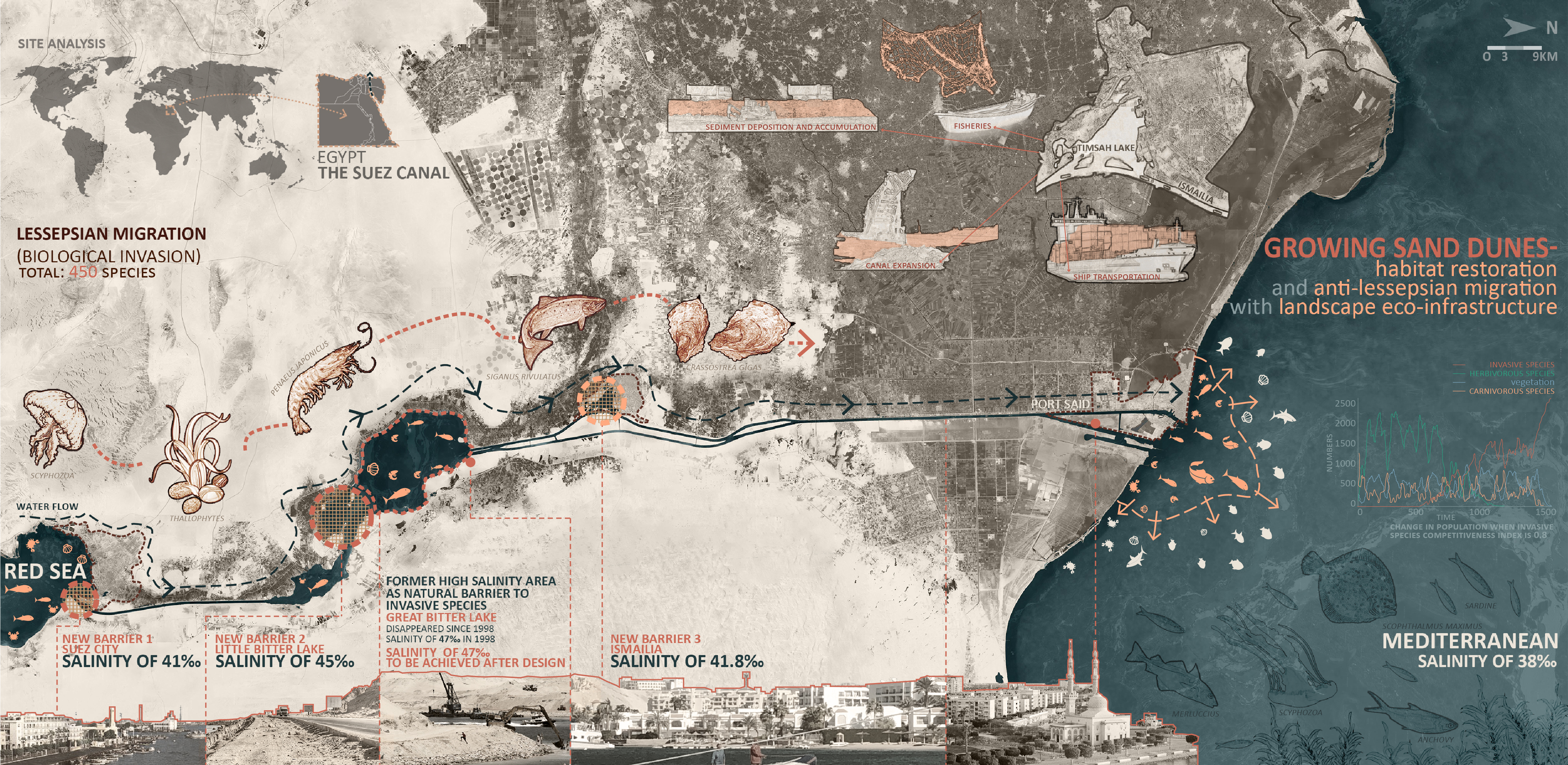This image is an old, beige and brown-toned map detailing the Lysippian migration, which refers to the biological invasion of about 450 species from the Red Sea to the Mediterranean Sea. The map specifically highlights key migration routes around the Suez Canal, situated near Egypt, and includes illustrations of various marine creatures such as shrimp, jellyfish, and fish to depict this invasive journey. Dark turquoise and blue colors illustrate the sea and ocean, showing where the species have invaded. Accompanying textual details, primarily in red, orange, and yellow, discuss "growing sand dunes," "salinity," "habitat restoration," and "landscape eco-infrastructure" — crucial elements of this migration story. Additionally, a white, colorless illustration of a city appears at the bottom, while a compass is placed in the top right corner. The map's annotations also refer to the Mediterranean's salinity level of 38%, enhancing the scientific context of the species' movement through this eco-network, culminating in their spread into the Mediterranean Sea.